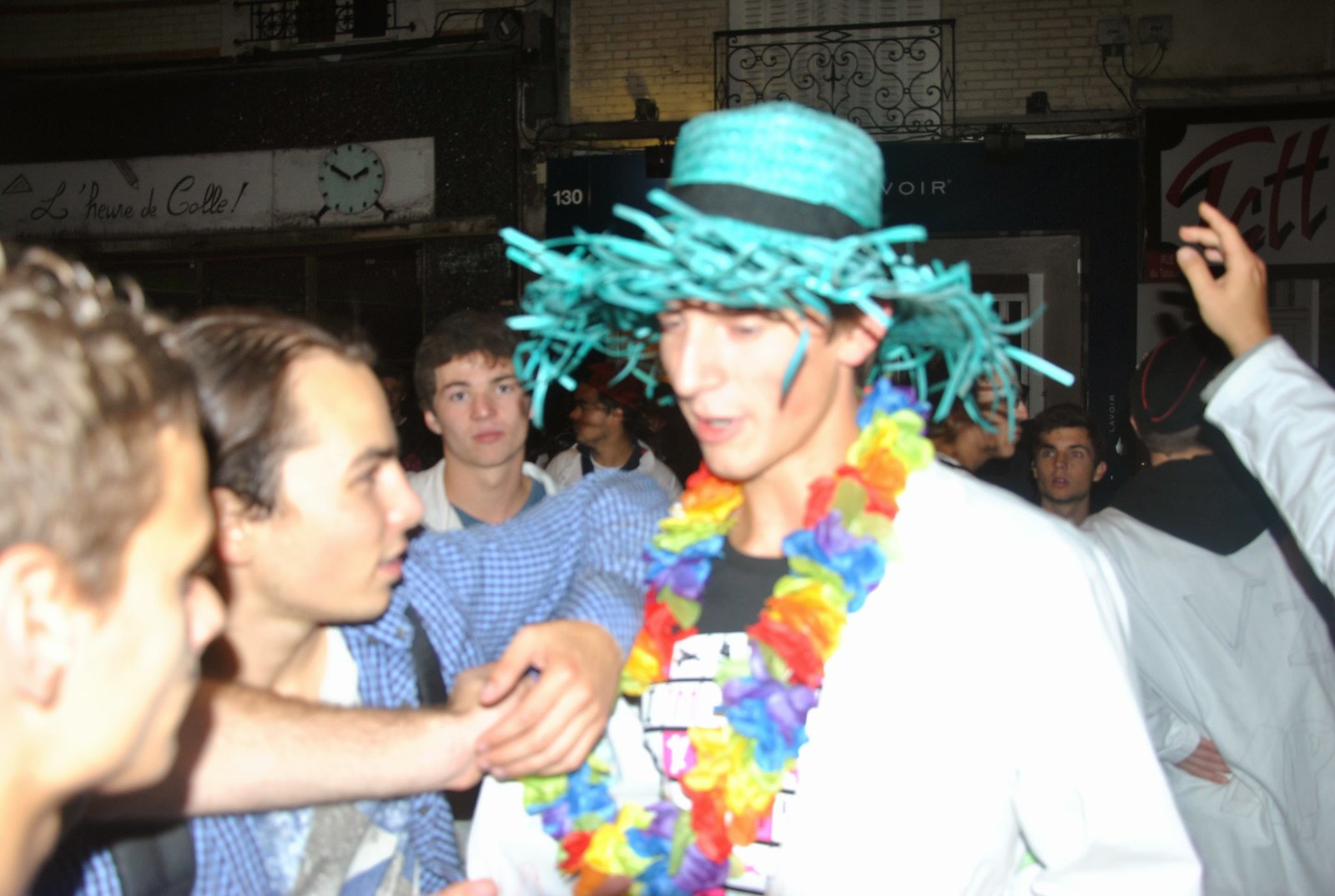The image depicts a scene that appears to be either at an outdoor nighttime event or possibly within a dimly lit bar. The central figure is a young man dressed in a white long-sleeve jacket over a black t-shirt that has some writing on it. He is wearing a distinctive blue straw hat, which is frayed around the edges and sports a black band. Alongside this, he has a plastic flower lei around his neck, typically associated with Hawaiian themes.

Standing to the right of him is another young man, dressed in a blue and white checkered button-up shirt. This person has their elbow resting on the main figure's left shoulder, and they seem to be engaged in an intense conversation. The setting around them is crowded, with several individuals visible in the background, some of whom appear to be in white gowns or robes. There are also buildings behind them, which suggests they're outside. Certain blurry signs in the background hint that the location could possibly be in France. The overall ambiance indicates a lively gathering, possibly a party or a festive celebration.